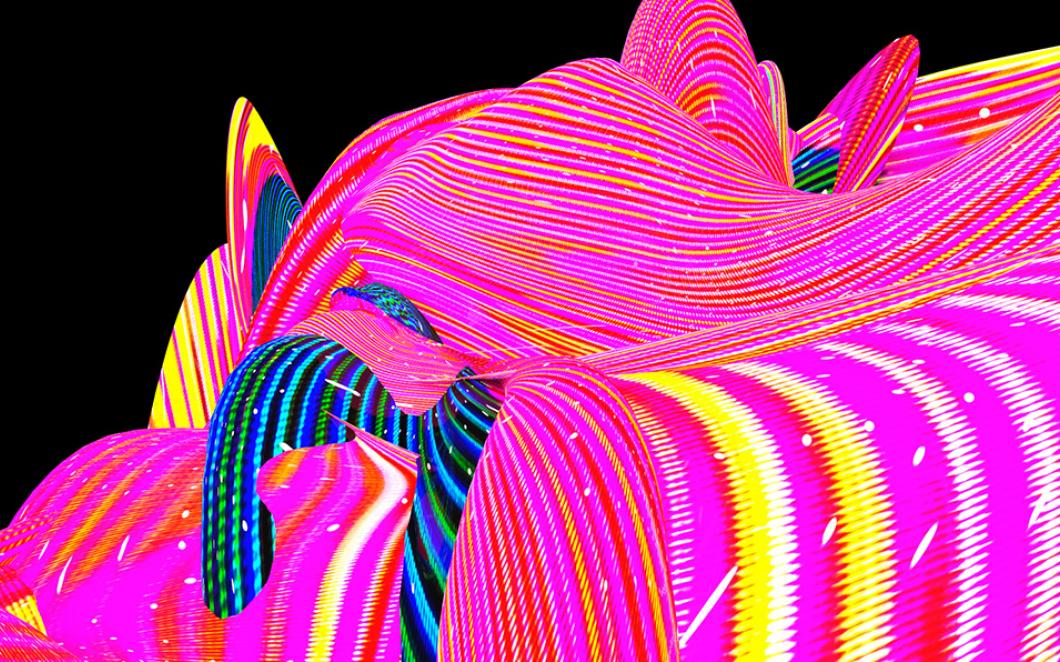This vibrant, neon-colored illustration showcases a dynamic play of hues and patterns. The background is predominantly black, creating a stark contrast that enhances the luminous quality of the image. The composition is primarily dominated by hot pink, with interwoven lines of yellow, red, and white creating a vibrant tapestry. These lines form swirling shapes and jagged line patterns, some resembling tiny X's, contributing to the overall energetic design. The top of the image features mostly horizontal lines, while the bottom half shifts to more vertical orientations. In the middle left, there's a striking section of dark blue fabric-like texture, interspersed with thin green and light blue stripes. This combination of colors and patterns, suggestive of neon lights, evokes a sense of joy and exuberance. The piece could be either hand-painted or computer-generated, but the exact technique remains ambiguous, emphasizing the abstract and modern nature of the artwork.